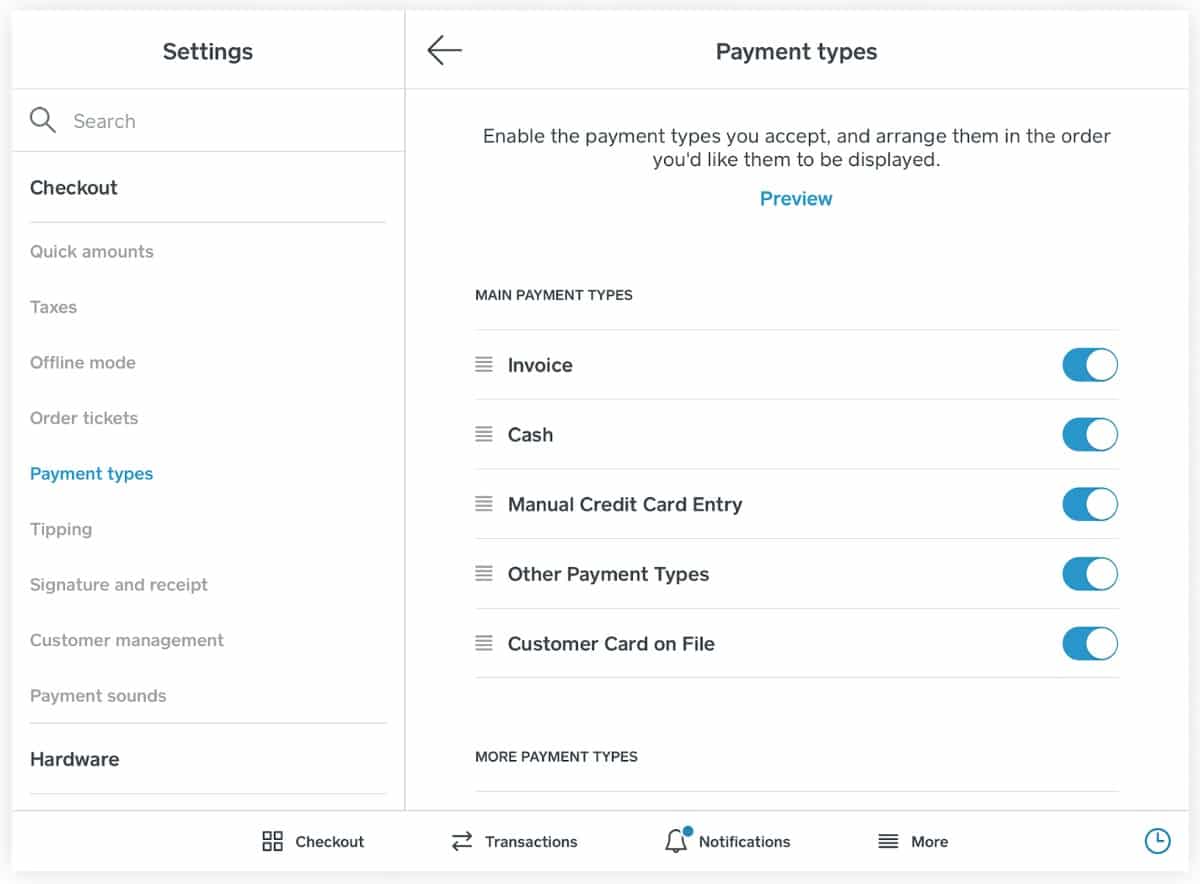The image displays a user interface primarily for configuring payment settings. On the left side, there's a menu box titled "Settings" which includes a search box adorned with a magnifying glass icon. Below this, there is a section labeled "Checkout" followed by a thin gray horizontal line.

The line segregates various settings options: "Quick Amounts", "Taxes", "Offline Mode", "Order Tickets", "Payment Types", "Tipping", "Signature and Receipts", "Customer Management", "Payment Sounds", and "Hardware."

On the right side, under the "Payment Types" section, there's an instruction: "Enable the payment types you accept, and arrange them in the order you'd like them to be displayed," along with a blue hyperlink for a preview. Beneath this, a list of payment methods is presented: "Invoice," "Cash," "Manual Credit Card Entry," "Other Payment Types," and "Customer Card on File." Each payment type has a toggle switch to its right for activation, colored blue to indicate an active status.

Further down, there's a section titled "More Payment Types," followed by options for "Checkout," "Transaction," "Notification," and a "More" button for additional settings.